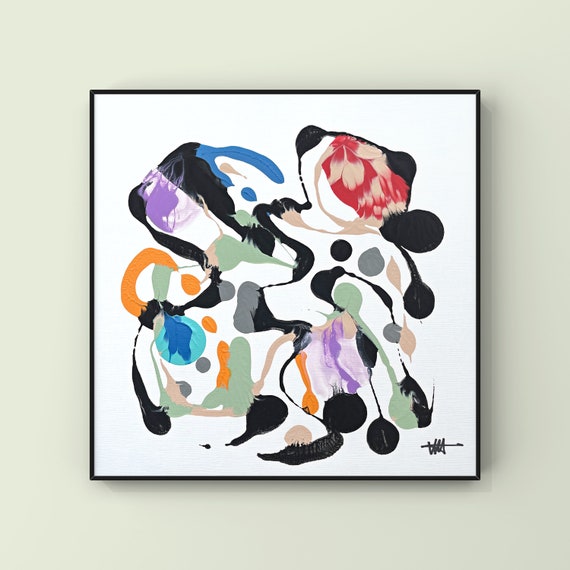This image depicts a modern abstract painting mounted on a white wall. The artwork is a white canvas bordered by a slim black frame. The painting features an assortment of black ink splotches, intermingled with blobs and strokes in vibrant colors, including shades of purple, blue, red, dull green, orange, and beige. The medium appears to be acrylic paint. These colorful elements are randomly distributed across the canvas, contributing to its abstract nature. The artist's signature, rendered in black ink, is located in the bottom right corner. The wall supporting the painting is also light beige, creating a subtle contrast with the white canvas.